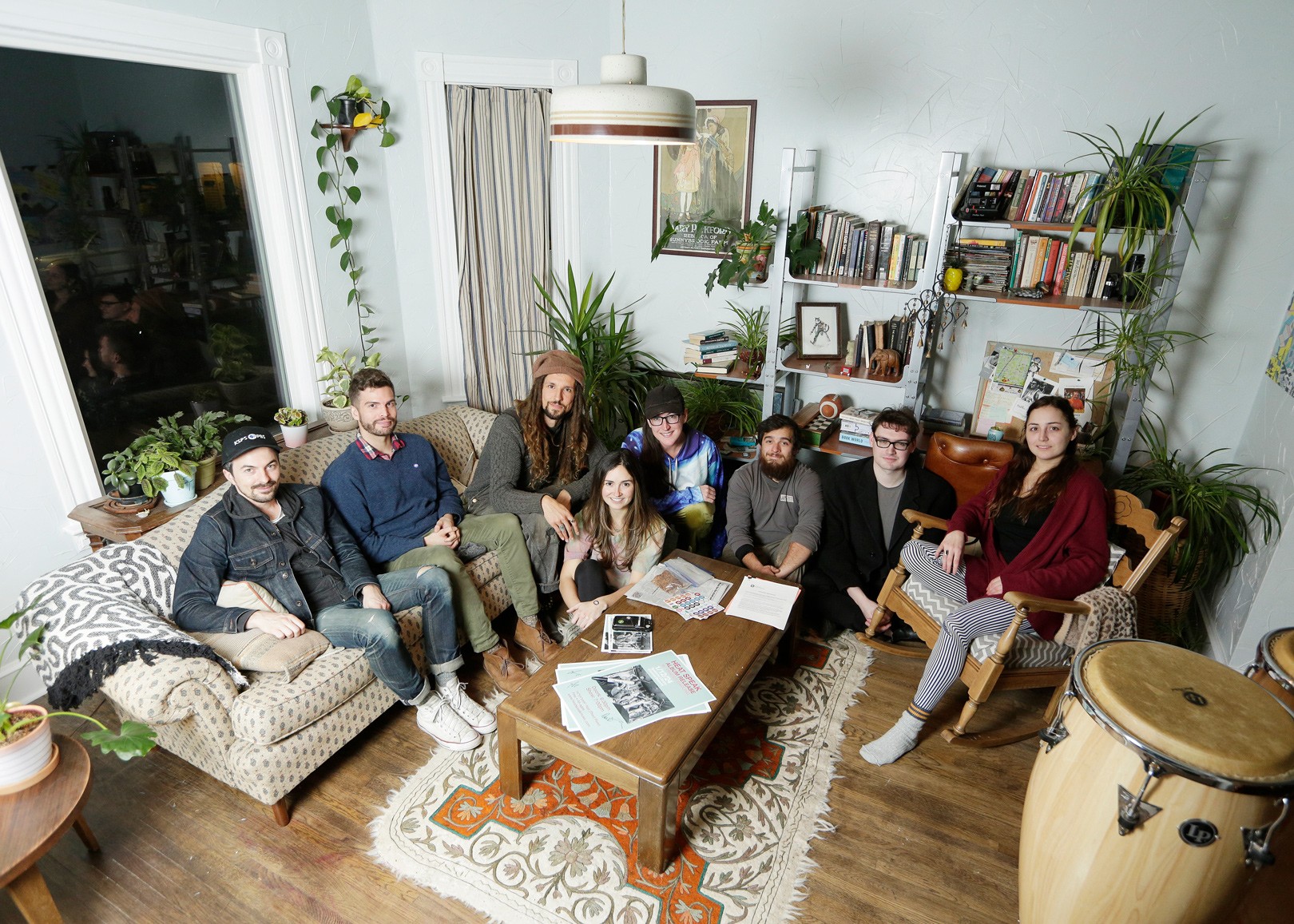In a brightly lit living room, a group of eight young adults, likely in their late 20s to early 30s, gather in a casual, artsy ambiance. The group, consisting of five men and three women, exudes a hipster or bohemian vibe, with many sporting jeans, beanies, and eclectic clothing. They are seated around a coffee table cluttered with newspapers and various papers, some on a beige-patterned couch adorned with a white blanket, others on chairs and the floor.

Prominently in the room are several plants, including a drooping vine and hanging greenery, giving the space a lush, organic feel. At the forefront are a set of brown bongos, adding to the creative atmosphere. Behind the group, there's a bookcase filled with a variety of books, indicating a love for reading or perhaps an intellectual flair. The backdrop also features a long vertical window draped with white embroidery, contributing to the room's bright and airy ambiance.

Among the individuals, detailed descriptions include a man in a jean jacket and ripped jeans, another in a blue ensemble and plaid shirt, a woman in a tie-dye shirt with black-rimmed glasses, and another woman in a multicolored shirt with black pants. Their relaxed postures and the casual arrangement of their seating imply a close-knit, friendly gathering, likely of friends or a community, enjoying each other's company in a warm and welcoming living room.